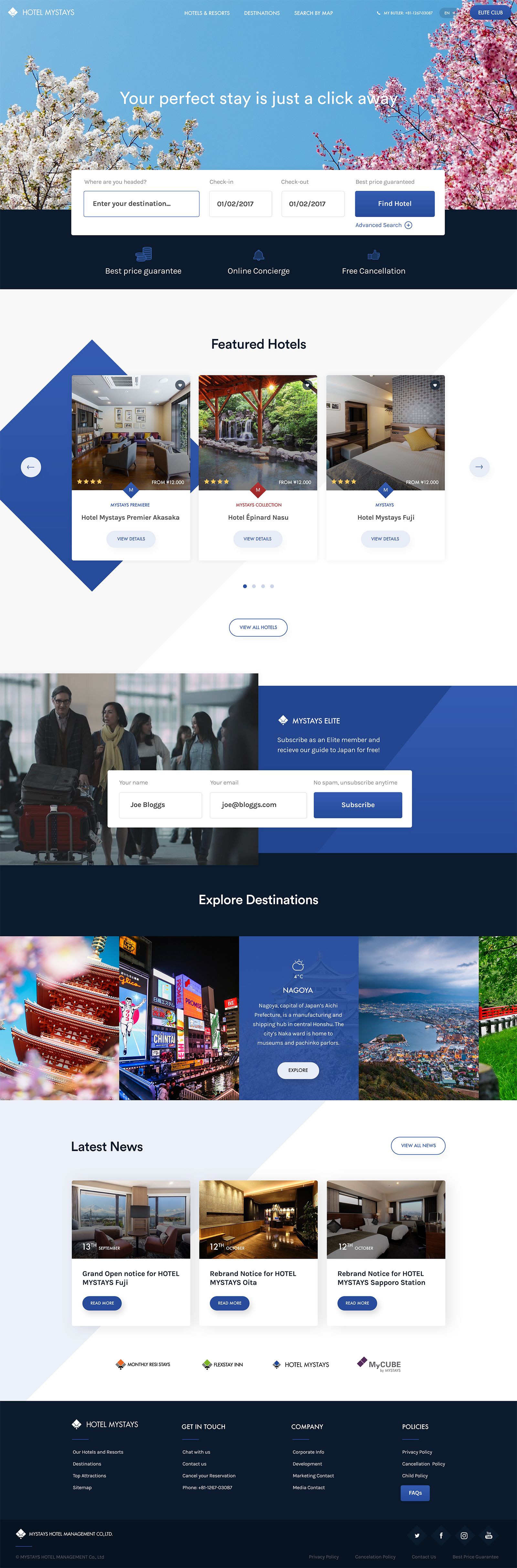The image appears to be a screenshot of the homepage for a travel website called Hotel My Stays. The site’s logo is prominently featured in the upper left corner. 

In the central section, the webpage offers three main navigation labels: "Hotels and Resorts," "Destinations," and "Search by Map." Positioned on the right side is the customer service contact information, labeled "My Butler," with the phone number +81-1267-03087, and an option for English language support.

The background of this upper section features a scenic view of Japanese cherry blossom trees, with the one on the left displaying whitish flowers and the one on the right showcasing pinkish blossoms. Across the blue sky between the trees, there's a welcoming message: "Your Perfect Stay is just a click away." Below that, in bold letters, it prompts users with "Where are you headed?" accompanied by a search box for inputting destinations. Details for "Check In" and "Check Out" default to 01-02-2017, suggesting placeholders for user-specific dates. Additionally, a "Best Price Guaranteed" message is displayed, with a prominent blue box labeled "Find Hotel" and an "Advanced Search" option underneath.

Following this section, a dark blue background is segmented into three horizontal sections highlighting various features: "Best Price Guarantee," "Online Concierge," and "Free Cancellation."

Beneath this, on a white background, is the "Featured Hotels" section showcasing three images. The first image likely depicts a living or entertainment room with couches and a possible TV on the left-hand side. The second image appears to be an outdoor scene, labeled "From 12,000." The third image shows a bedroom also labeled "From 12,000." Detailed information for these featured hotels reads:
1. My Stay's Premier, Hotel My Stay's Premier, Alaska, with a "View Details" button.
2. My Stay's Collection, Hotel Epinard Nassau, with a "View Details" button.
3. My Stay's Hostel, My Stay's Fuji, with a "View Details" button. All hotels boast a four-star rating.

Below the featured hotels, there's a blue-bordered oval button labeled "View All Hotels." 

Further down, another section features an image of travelers at an airport. To the right, it reads "My Stay's Elite," encouraging visitors to subscribe as an Elite member to receive a free guide to Japan. Input fields for "Your Name" and "Your Email" (e.g., Joe Blogs and joe@blogs.com) are provided, along with assurances of "No Spam" and the option to "Unsubscribe anytime," culminating in a "Subscribe" button.

An "Explore Destinations" segment follows, displaying various scenic locations in Japan. One highlighted block features Nagoya, with a temperature reading of 4 degrees Celsius. A brief description notes, "Nagoya, capital of Japan's Aichi Prefecture, is a manufacturing and shipping hub in central Honshu. The city's Naka Ward is home to museums and pachinko parlors," along with an "Explore" button.

The "Latest News" section lists headlines and dates:
1. "Grand Open Notice for Hotel My Stay's Fuji, 13th September."
2. "Rebrand Notice for Hotel My Stay's Oita, 12th October."
3. "Rebrand Notice for Hotel My Stay's Sapporo Station, 12th October." A "View All News" link is provided on the right.

At the bottom of the page, sections labeled "Monthly Resi Stays," "Flex Stay In," "Hotel My Stays," and "My Cube" are displayed.

Altogether, the image illustrates the comprehensive and inviting design of the Hotel My Stays website, providing users with a range of options and information for planning their stays.